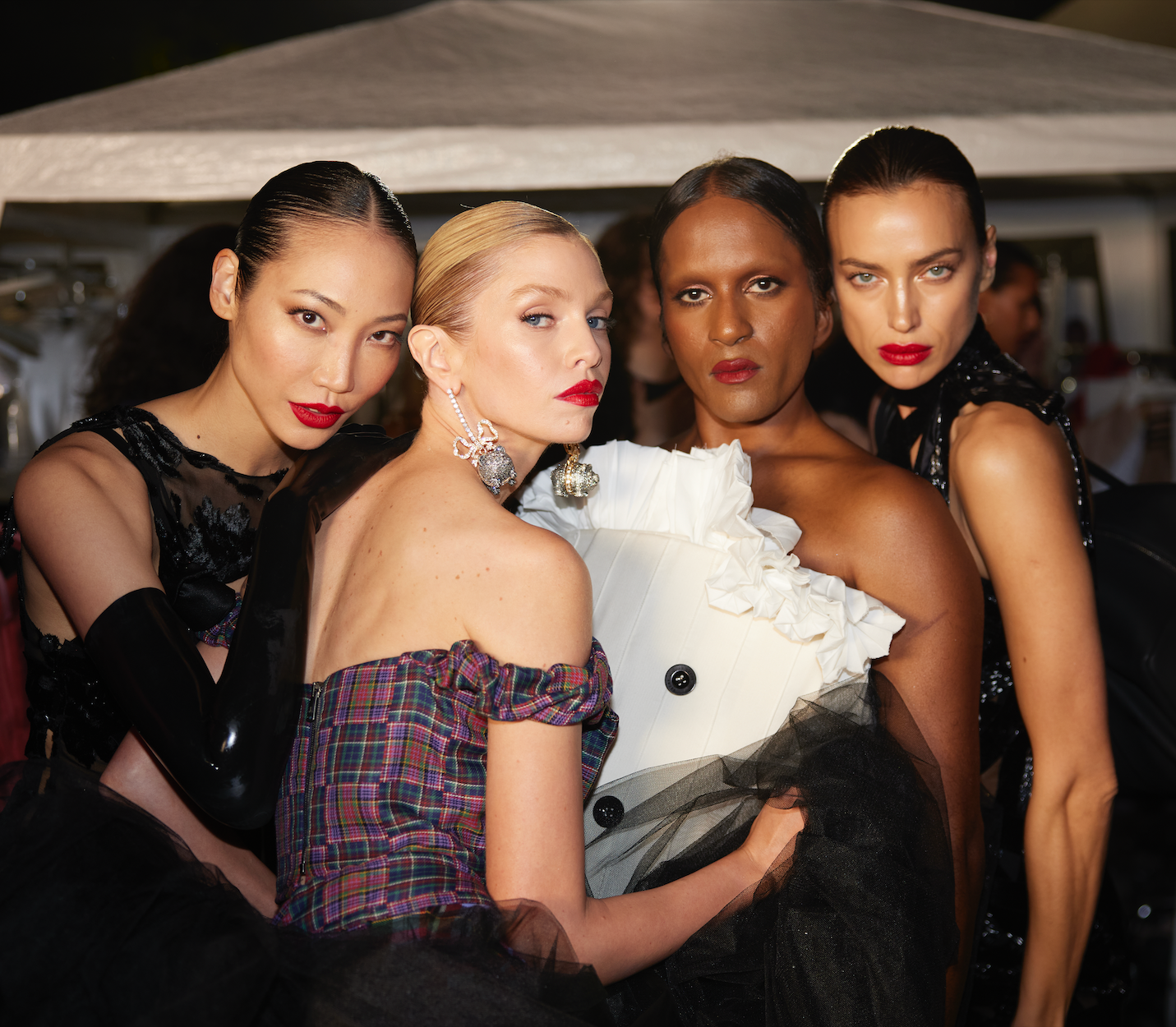This photograph features a close-up of four models standing closely together, all looking directly at the camera with serious expressions. The two individuals on the left appear to be presenting as female, with the far-left person being an Asian woman, identifiable by her pulled-back hair styled in a bun, and wearing a black, gauzy, shoulderless dress, complemented by a black glove on one hand. Beside her is a blonde woman with silvery, dangling earrings that resemble a series of linked circles, or possibly a necklace, and she dons a plaid dress with shades of purple and pink that sits off her shoulders. The third model from the left has dark skin, suggesting potential African-American heritage, and wears a distinctive white, frilly top, although part of their outfit is obscured by an object held by the blonde. Finally, to the far right is another individual with black hair pulled back, dressed in a black outfit. The gender presentation on the right side is less clear, possibly indicating these individuals are gender non-conforming or in drag. All four share the common feature of bright red lipstick. In the background, there are people milling about under a white overhang, possibly suggesting an event or booth setting.